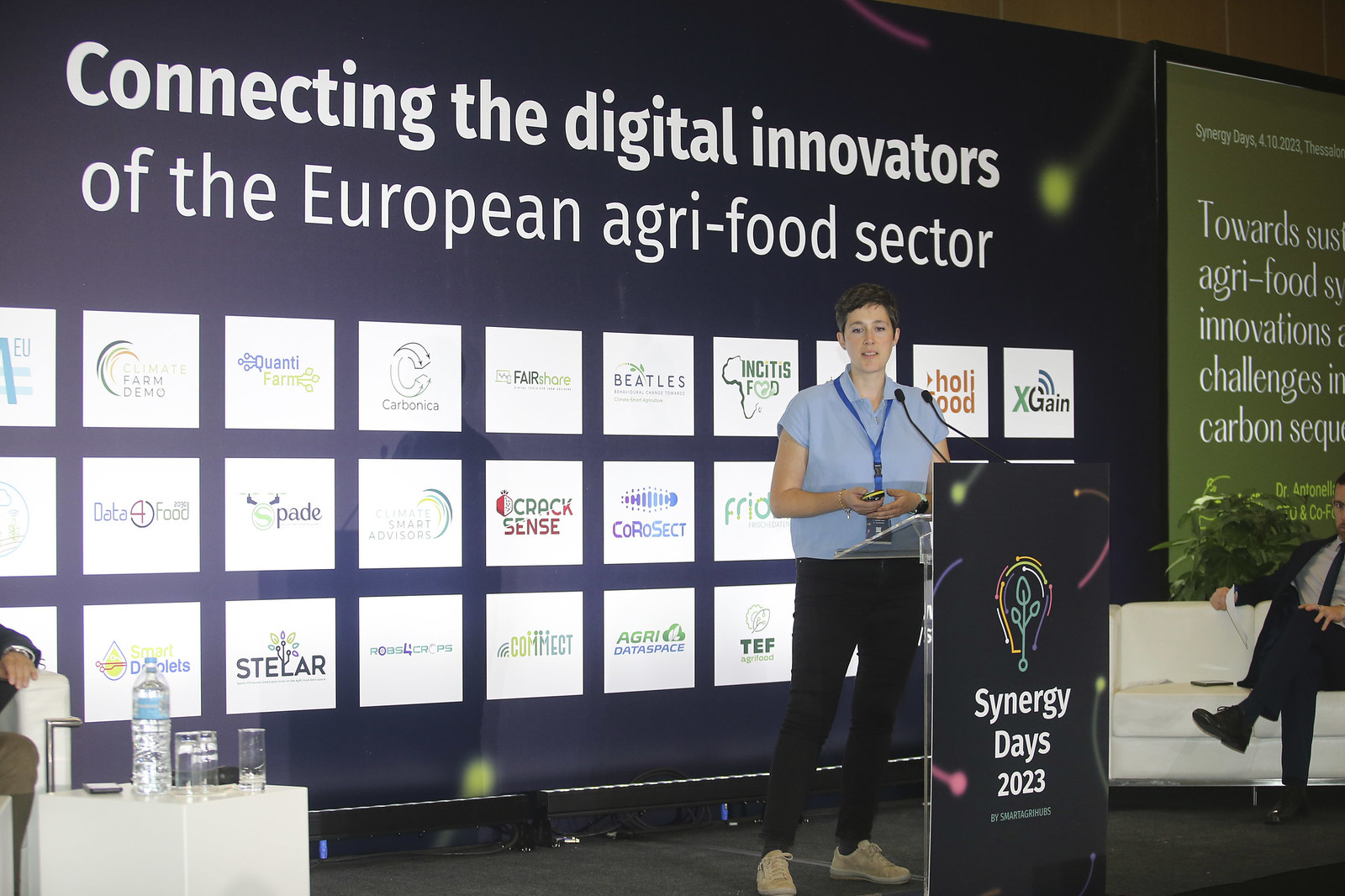In this image, a woman with short brown hair stands behind a podium adorned with a black sign reading "Synergy Days 2023." The sign features an artistic rendering of a multi-colored lightbulb with a plant inside, surrounded by swirling comet-like designs. The woman is dressed in a short-sleeved blue shirt, black pants, and white shoes, with a blue lanyard and picture ID hanging near her navel. She appears to be giving a speech on a small, elevated black stage.

Behind her, a large digital screen displays the text "Connecting the Digital Innovators of the European Agri-Food Sector" in bright white letters against a navy blue background. The screen is filled with rows and columns of white boxes, each showcasing various company logos.

To her left, the right of the image, a man in a dark blue suit with a white shirt and blue tie sits on a white couch, which is accompanied by a green sign partially obscured but suggesting a focus on sustainability in agri-food innovations and carbon sequestration. Further to the left, there is another seating area with a white couch and a white cubed coffee table, topped with bottled water and glasses. A man's hand, wristwatch, and khaki-colored pants are partially visible in this section of the image. The setting appears to be an indoor business center, with a general atmosphere of a professional conference or seminar.